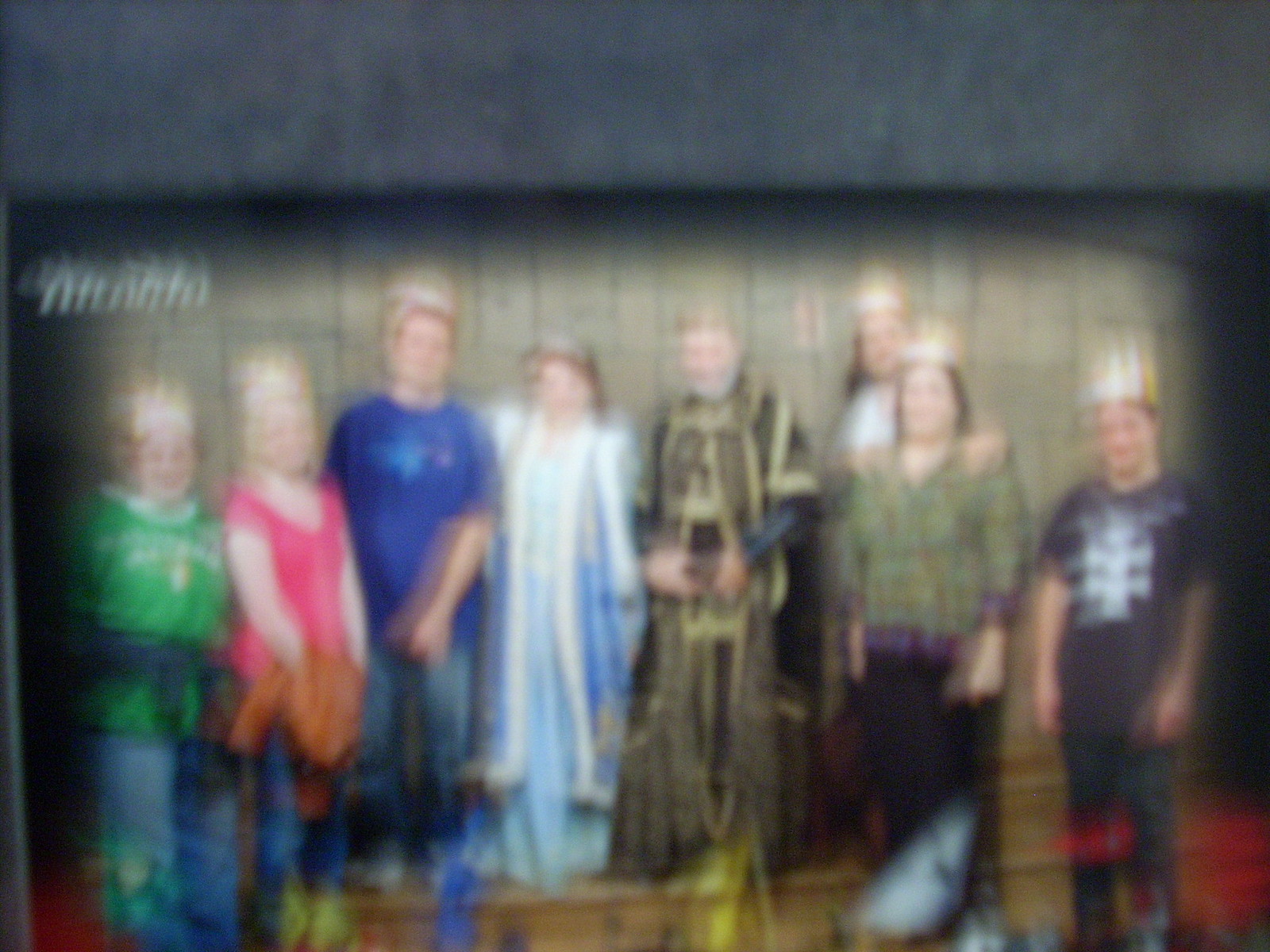A vintage, slightly blurry photograph captures a close-knit family moment, possibly during a Halloween season. The group consists of eight people, predominantly children, with a mix of costumes adding a playful element to the scene. Two of the younger members are clearly in Halloween attire, one notably wearing a crown. The presence of a parent is discernible, as a young girl clings to her mother in the background, suggesting familial warmth and connection. The photo's setting and a subtle, indistinct timestamp hint at a classic JCPenney's photoshoot, evoking a sense of nostalgia. This intimate and casual family gathering is beautifully captured despite the image’s lack of sharp clarity.